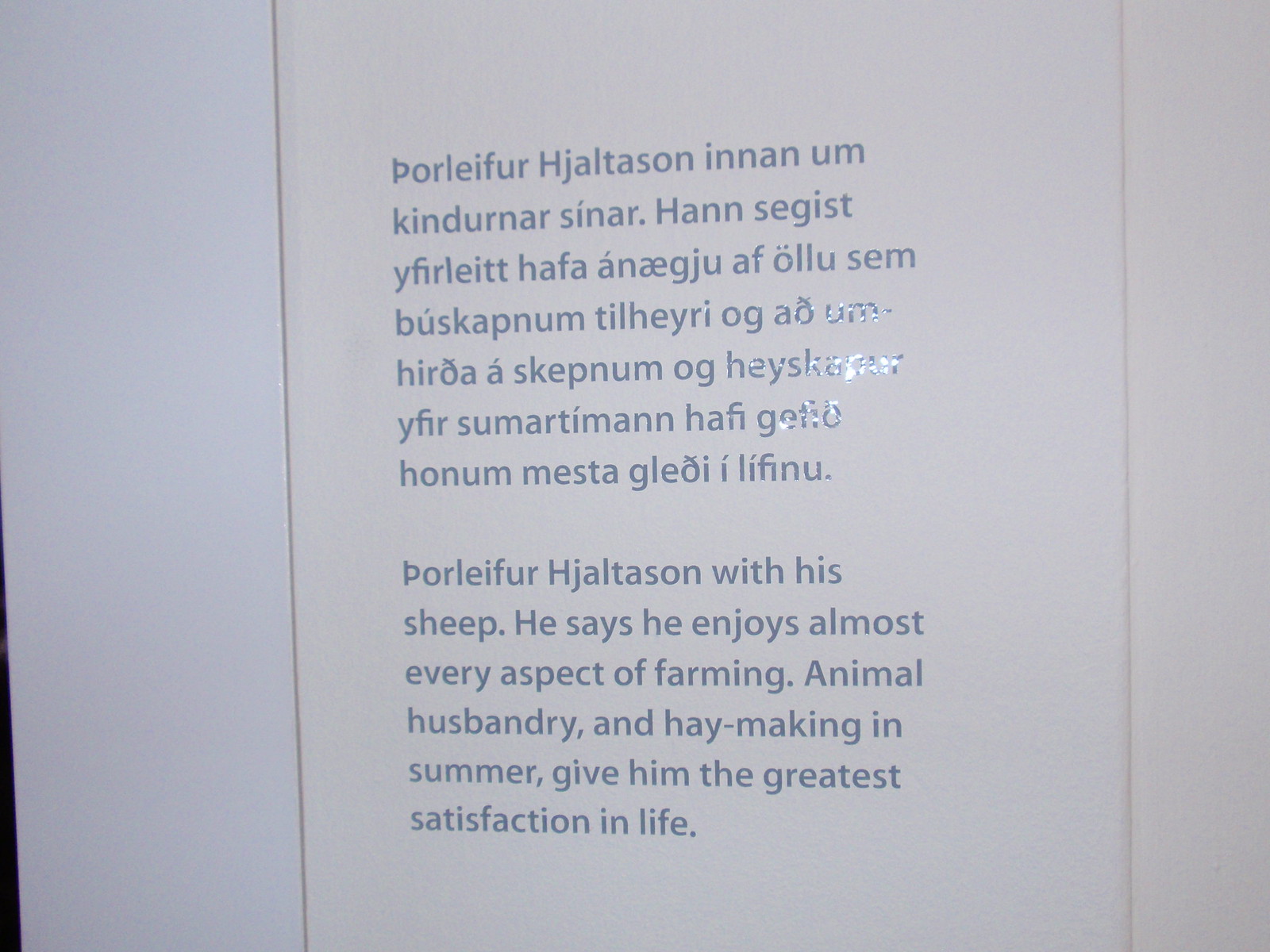The image depicts a framed panel resembling a torn-out page from a book. The page features two paragraphs: the top paragraph, written in a language unfamiliar to the describers, spans approximately seven lines. The bottom paragraph is the English translation, stating, "He says he enjoys almost every aspect of farming. Animal husbandry and haymaking in the summer give him the greatest satisfaction in life." The text is in light blue font on a white background, with a very thin gold stripe around the edge. Additionally, there is a small black area and a light blue border on the left-hand side.